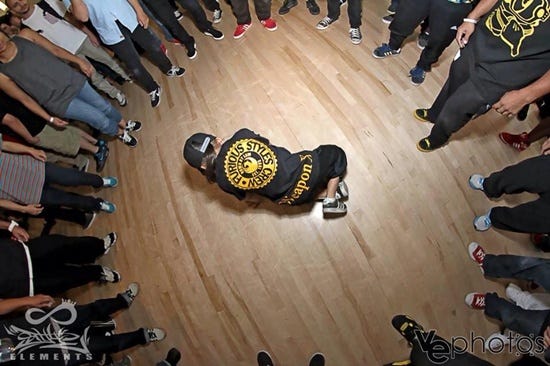This overhead image captures a dynamic scene of a large group of people, possibly middle school-aged or early teenagers, gathered in a perfect circle on a hardwood floor, suggesting a dance group or community event. Most of the people wear casual black pants or blue jeans, along with a variety of sneakers in colors such as red, red and white, black and white, and blue and white. A notable detail is the sole individual in the center of the circle, laying on their side or stomach, potentially breakdancing. This person is dressed in a black shirt with a yellow emblem and text that reads "Furious Styles Crew." The person also wears black pants, black and white sneakers, and a baseball cap. The bottom left of the image has the word "elements," while the bottom right reads "VE photos." The photo is taken from directly above, contributing to the unique perspective mostly showcasing legs and feet, adding to the mystery and energy of the scene.